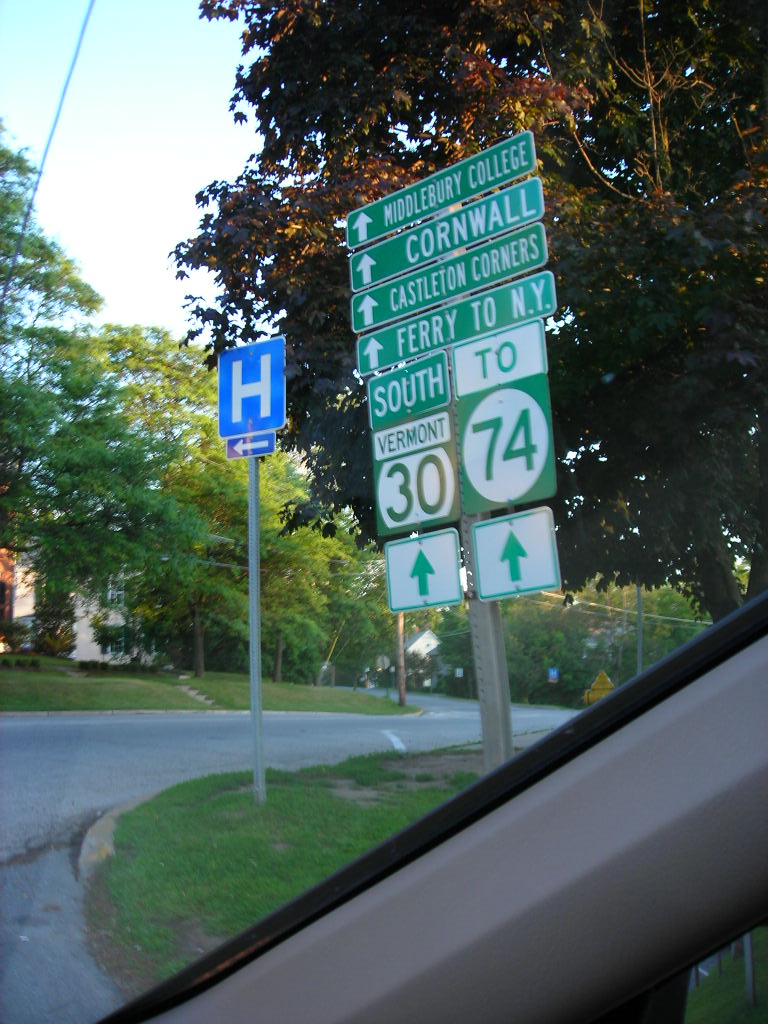The image shows a bustling street corner in a residential area, taken from inside a car through the front windshield. Dominating the scene is a large metal post featuring multiple signs pointing in various directions. At the top, a green sign lists four destinations with arrows pointing north: Middlebury College, Cornwall, Castleton Corners, and Ferry to New York. Flanking both sides below are additional signs: one on the left indicating "South Vermont 30" and one on the right for "Route 74." A blue square sign with a white "H" and an arrow points left, signaling the direction to a nearby hospital.

The roadway is gray and crosses from left to right just below the center of the image. Off to the left side, partially obscured by grass, is the edge of a fire hydrant. The background includes lush green trees and a few residential houses, further suggesting a small-town or suburban setting. The sky above is clear and blue, enhancing the outdoor, sunny ambiance.